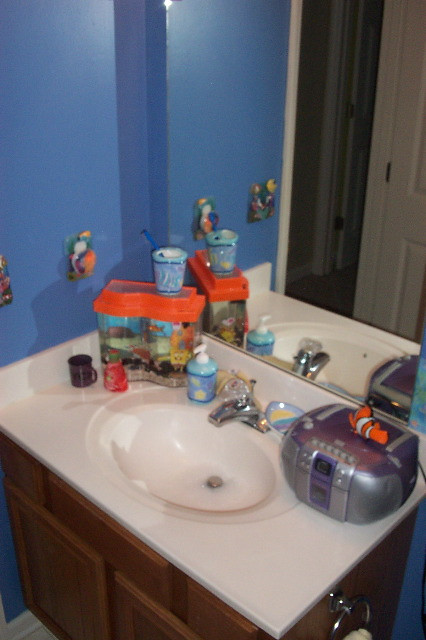This photograph captures a retro bathroom scene prominently featuring an integrated sink and countertop from the 1970s. The vista, reflected in a large wall-mounted mirror above the sink, offers an expansive view of the vanity area. The sink is equipped with a classic single-knob faucet. Nestled in the upper right-hand corner of the sink is an old CD boombox, hinting at the era of the setting. Below the sink, a wooden cabinet sports a small towel rack. On the right side of the sink countertop, there is a push-down hand soap dispenser, a small black cup, and a ceramic container that doubles as a toothbrush holder, identifiable by its multiple holes designed to hold toothbrushes and toothpaste. A mysterious red container also rests on the sink, its purpose unknown within the context of the image. This detailed snapshot invites the viewer to step back into a bygone era with its vintage charm and character.